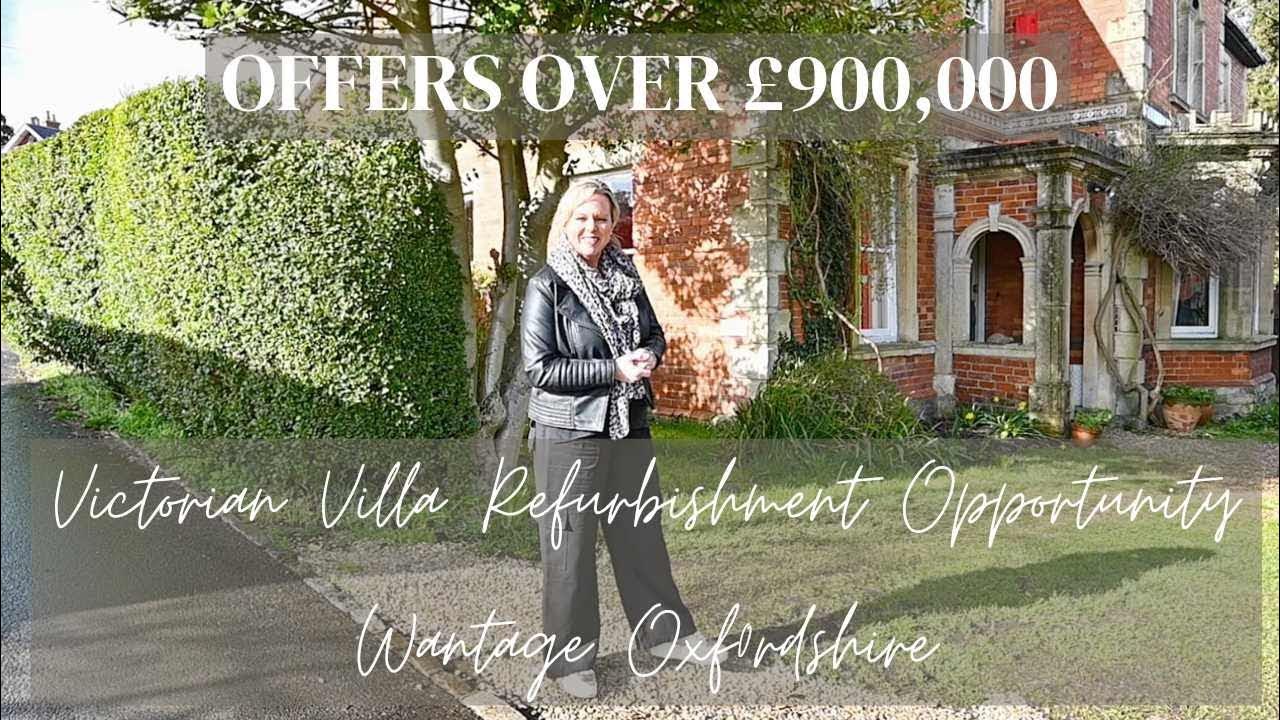A horizontally aligned rectangular picture captures a woman standing on a neatly maintained lawn near a sidewalk, situated in the lower left corner. She is smiling directly at the camera, her short, shoulder-length blonde hair parted, dressed in a black leather jacket over a cheetah print scarf, gray wide-leg pants, and white tennis shoes. Her hands are clasped together. 

In the background on the right side, there is an older, two-story Victorian brick house, constructed from a mix of red and white stone, whose façade is adorned with vines climbing up in different areas, contributing to its aged appearance. The house seems to be in a state that suggests a need for refurbishment. To the left of the house stands a sparse-leaved tree, likely a birch. Further left near the tree, a tall, approximately 12-feet-high hedge fence runs along the yard, creating a natural barrier between the yard and the road. Various flower pots are placed in front of the house, adding a touch of homeliness to the scene. 

Above the image, bold white letters read "OFFERS OVER £900,000" and at the bottom, in white cursive, it states "Victorian Villa Refurbishment Opportunity, Wantage, Oxfordshire." The sky above is partly cloudy, suggesting a sunny day with some clouds scattered around.